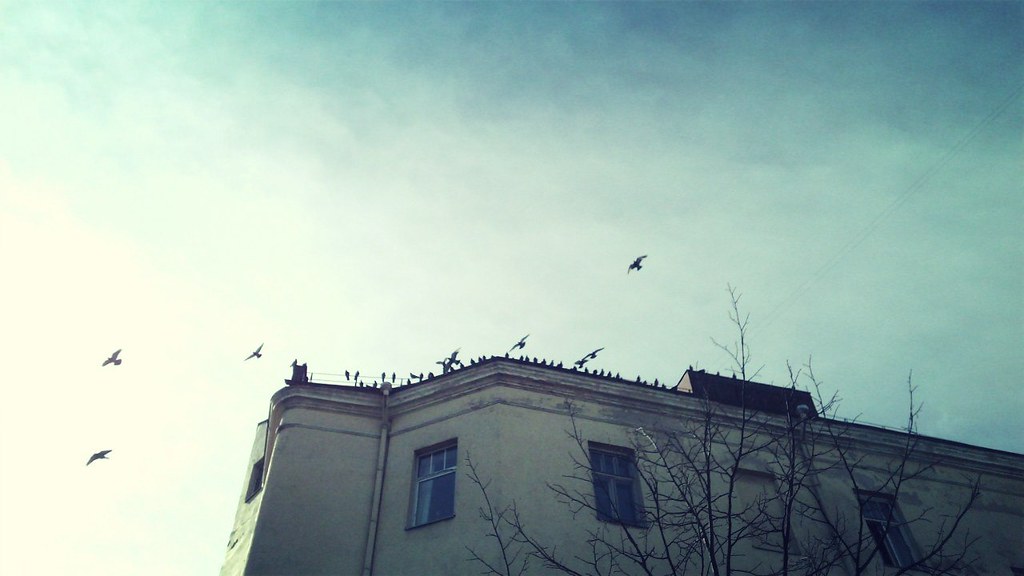This artistic and moody photograph, likely edited with Photoshop or a vignette filter, captures the top floor of an old-fashioned, sparse concrete building framed by a bare tree's branches. The image, taken from ground level, shows no text and features about 30 to 40 pigeons densely perched along the edge of the roof, with several more birds captured mid-flight against a semi-bright, bluish-tinted sky. The building's facade, predominantly white and unadorned, includes residential windows, some with curtains, suggesting it may now be converted into apartments. The lighting emphasizes a dramatic contrast, with the bottom left of the frame being very light and the top right fading into darkness, adding to the photograph's atmospheric quality.